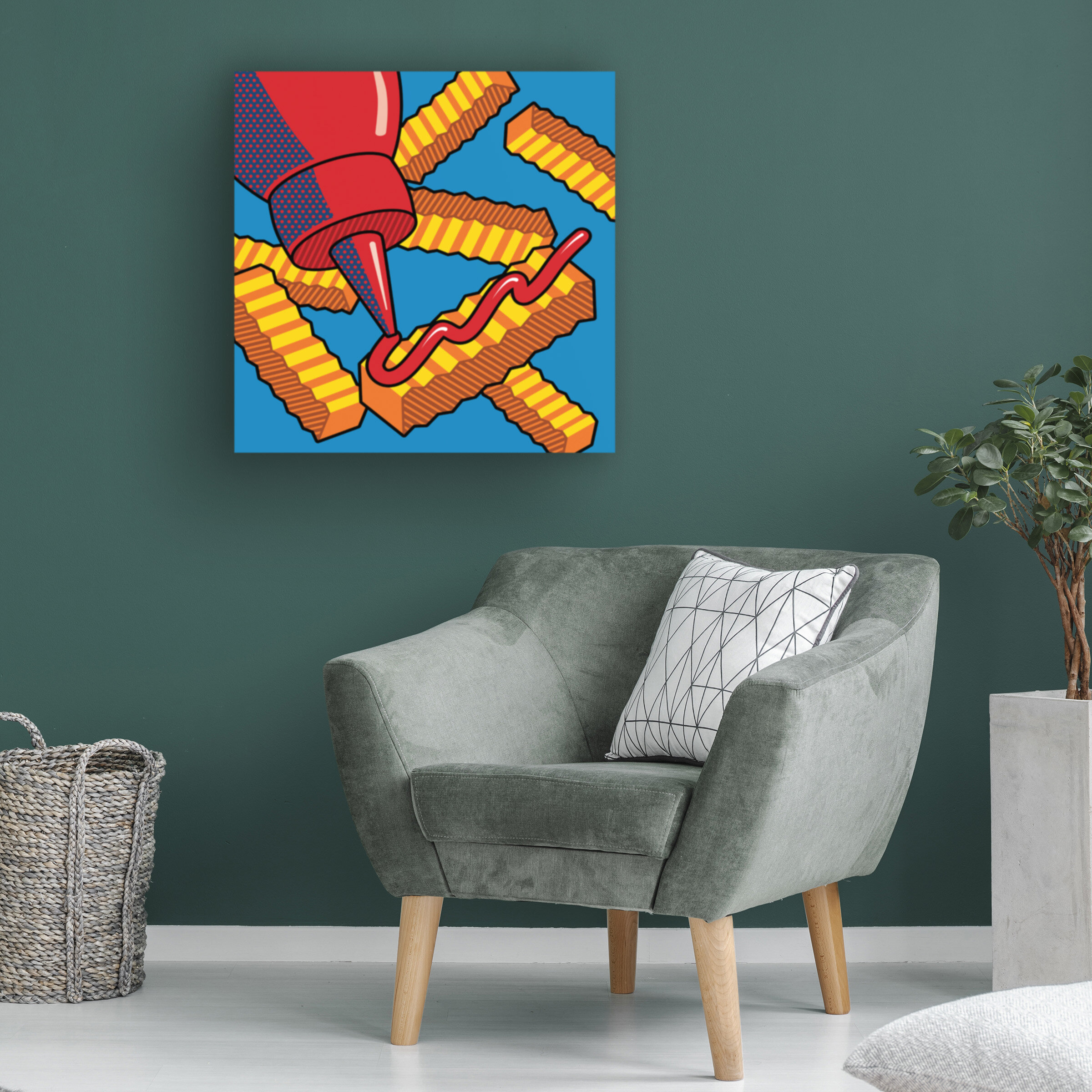The photograph depicts a stylish and modern room characterized by its cohesive color scheme and eclectic art piece. The focal point is a low, gray suede chair with teak legs, adorned with a white pillow featuring a gray line crisscross pattern. This chair sits against a deeply-hued blue-green wall, adding a contemporary but cozy atmosphere to the space. Mounted above the chair is a vibrant, comic book-style canvas showcasing a red ketchup bottle squirting ketchup onto floating crinkle-cut fries, which stands out dramatically against the otherwise neutral setting. To the left of the chair sits a dark gray wicker basket on the gray floor, while to the right, a gray rectangular table holds a white planter with a lush, green jade plant. The room’s elements blend modern aesthetics with playful artwork, creating a visually engaging yet comfortable environment.